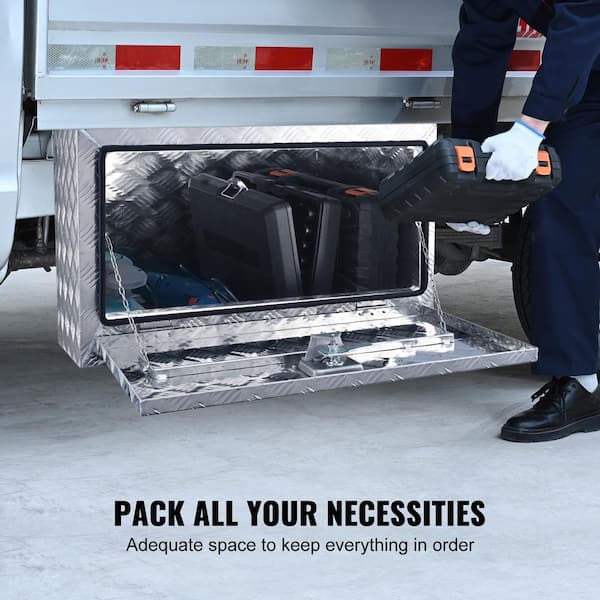The image appears to be a realistic photograph styled as an advertisement for a sturdy storage compartment designed for a utility vehicle. The compartment is constructed from stainless steel, suggesting durability and weatherproofing, and is located at the bottom or side of a white truck. The truck itself is mostly out of view, with only hints of its structure visible, such as red and white reflector strips.

In the right-hand side of the image, a man dressed in dark navy overalls, white gloves with blue trimming, and black dress shoes is seen in a crouched position, inserting a small black suitcase into the cargo space. The man’s upper body remains cropped out of the frame, focusing attention on his actions and the storage unit.

The cargo area door is open, supported by chains, revealing an organized interior with multiple small suitcases and a blue item. A notable feature is the reinforced and lockable design of the compartment, emphasizing security and practicality.

Text at the bottom of the image reinforces the marketing message: "Pack all your necessities, adequate space to keep everything in order." This suggests ample storage capacity and organizational benefits, making it a valuable accessory for professionals in need of a robust and reliable storage solution.